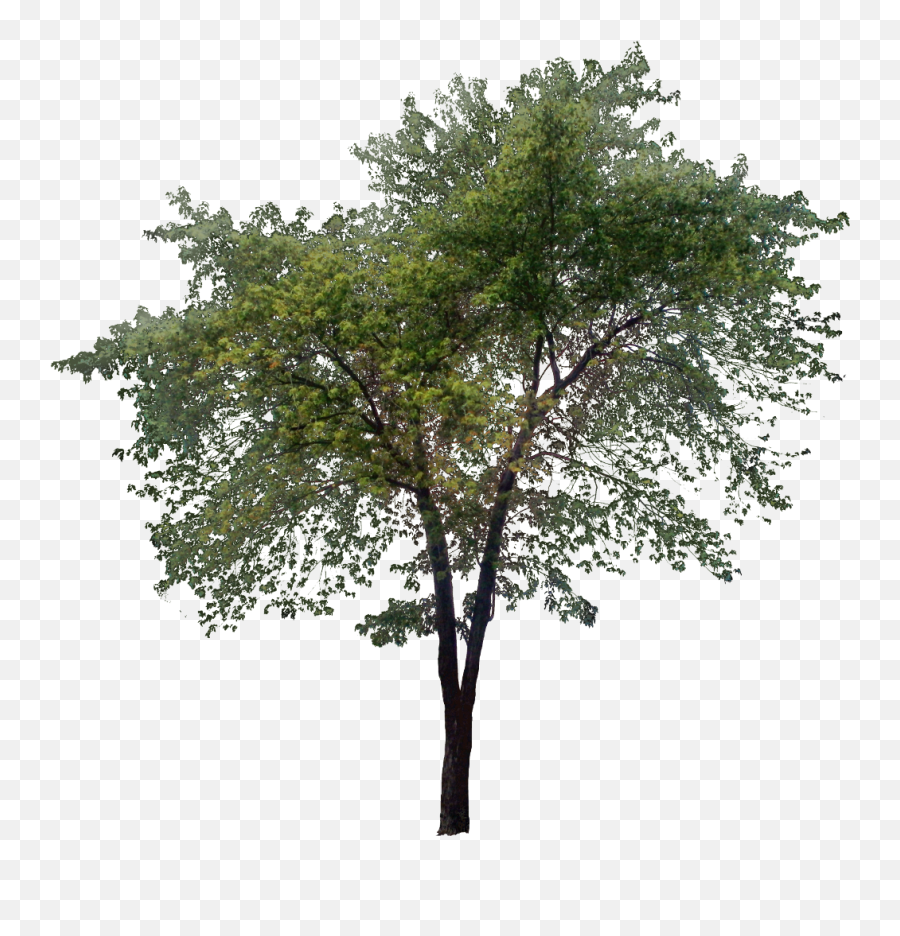The image features a tall tree with a dark brown trunk that appears almost black at its base, gradually lightening as it ascends into the branches. The trunk is sturdy and thick at the bottom, splitting into two main branches about 20% of the way up. These primary branches continue to fork into smaller ones as they extend upwards. The tree is adorned with an abundance of green leaves, which are particularly vibrant and reminiscent of spring or summertime foliage. A notable detail is that the leaves start about 30% up the tree and cover it entirely to the top, with some leaves appearing slightly lighter towards the middle left section.

The tree is set against a plain, checkered background composed of alternating white and gray squares, creating a grid pattern that spans the entire backdrop. This setting makes the tree appear as if it is suspended in the grid, emphasizing its centered positioning within the frame. The overall composition highlights the natural beauty and detailed structure of the tree, juxtaposed against the stark simplicity of the geometric background.